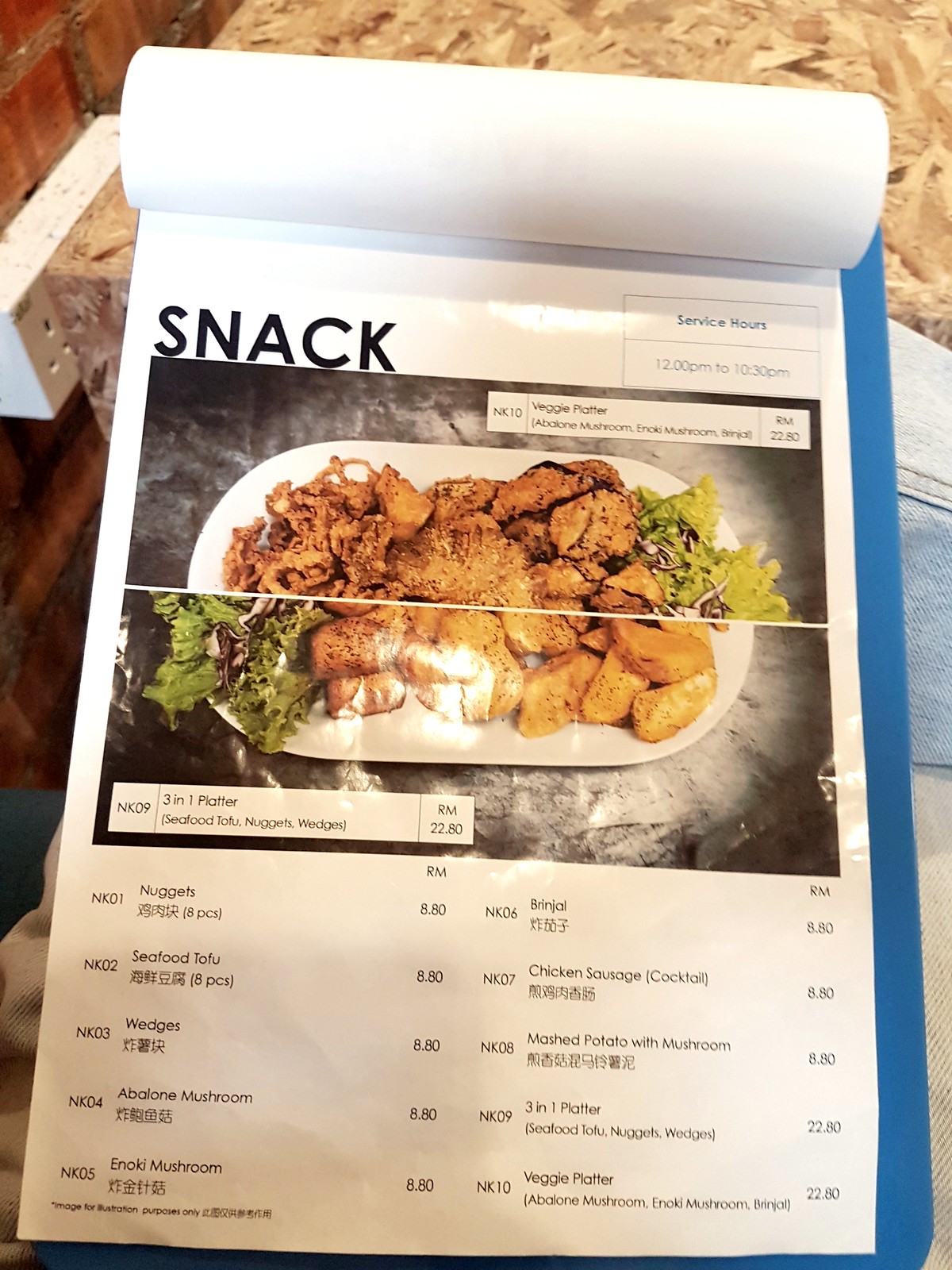The image depicts a menu attached to a clipboard with a blue background. The menu's heading, written in black font, reads "Snack." In the upper right corner, the service hours are listed as 12 p.m. to 10:30 p.m. At the center of the menu is a slightly blurry image of a veggie platter. Below this, clearer text describes a "Three-in-One Platter" that includes seafood, tofu, nuggets, and wedges. Additional individual menu items are listed, including nuggets, seafood, tofu, wedges, abalone mushroom, enoki mushrooms, brinjal, and chicken sausage (noted as "cocktail" in parentheses). There is also an option for mashed potato with mushroom, alongside the three-in-one platter and veggie platter. The menu contains some characters in a language other than English.